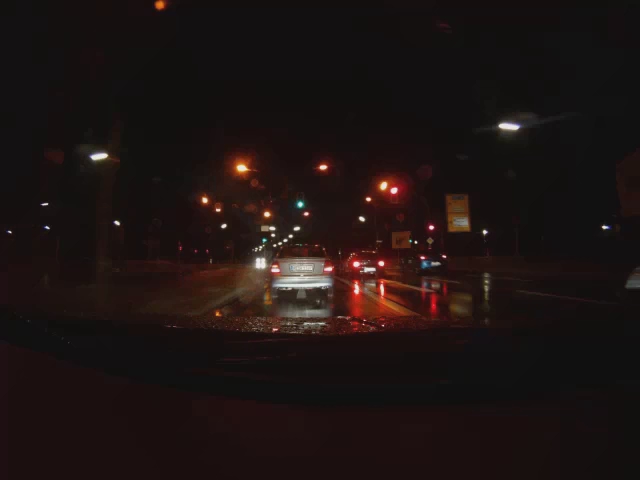A nighttime scene captured from within a vehicle showcases a wet road glistening under various lights. In the foreground, a silver car is visible, identified by its illuminated taillights on the right-hand side. The road stretches ahead with a series of red and green lights from traffic signals leading into the distance. Further down, yellow streetlights flank the road on both sides, casting their glow onto the moist pavement. A sign is faintly visible in the background, adding context to the urban setting. The reflective surface of the road mirrors the array of colors from the lights, emphasizing the dampness of the night. The overall atmosphere is serene yet bustling, characteristic of a vibrant city after rainfall.